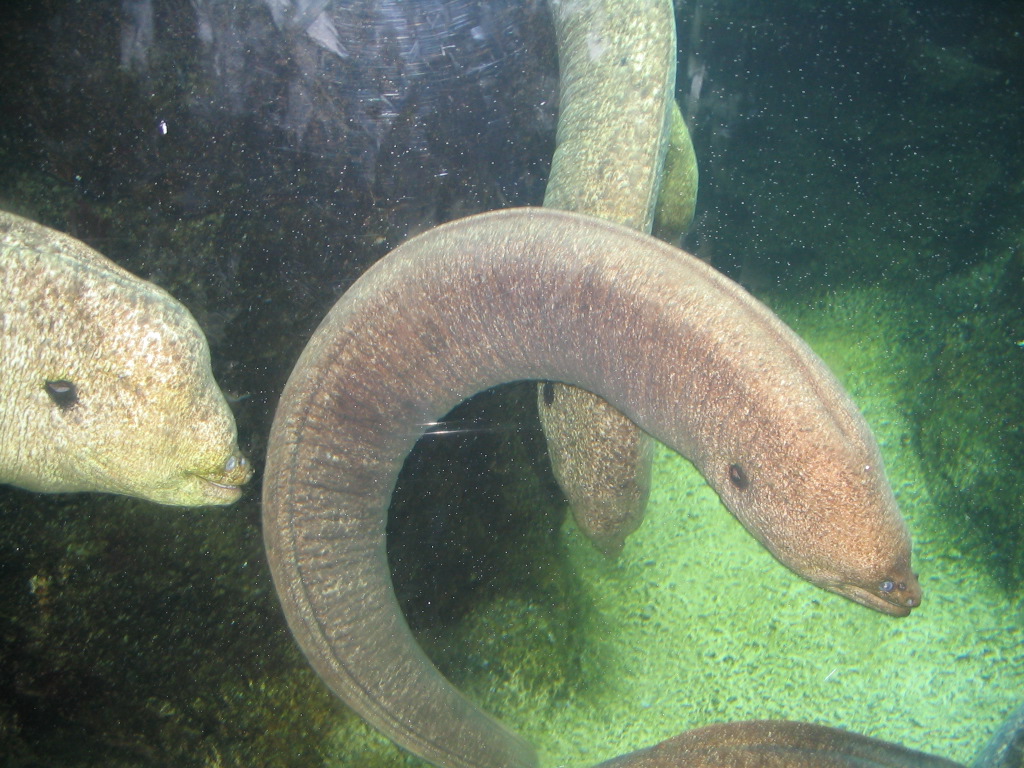In this detailed photograph taken at an aquarium, three moray eels are featured prominently, viewed through a pane of glass which shows small dots and fine lines indicative of the barrier. The eel closest to the viewer is intricately curled in a horseshoe or C shape, with its grayish-brown body marked by lighter yellow and white specks. This eel has striking blue eyes with black irises, and a darker circular spot resembling an ear. Positioned behind it, another eel of lighter tan hue also exhibits white specks on its body. Towards the left side of the image, a different type of fish with a white and dark tan speckled pattern and a prominent black circular mark is visible. In the backdrop, the aquarium scene is completed with greenish rocks and aquatic vegetation, creating a naturalistic habitat for these fascinating creatures.